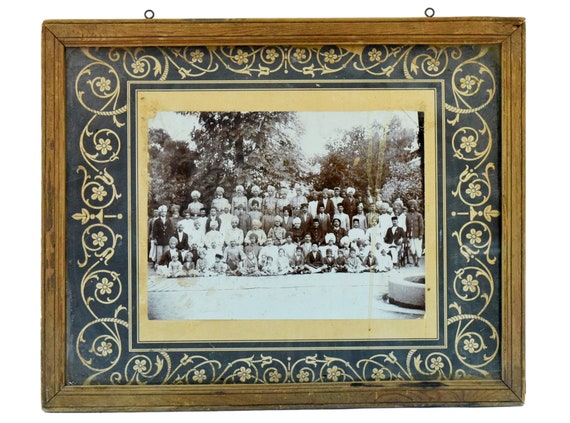The image depicts an intricately framed, vintage black-and-white photograph likely from the late 1800s, showing a large group of men in traditional attire. The rectangular frame is crafted from light brown wood, detailed with natural grain patterns, and has two black, circular hanging loops at the top. Encasing the photograph is an ornate pattern of yellow swirls and flowers set against a dark navy blue or greenish-blue background, forming a decorative border. Inside this border, a yellow rectangular area further frames the photograph. The scene captures approximately four rows of men, with those in the front rows seated, including children, and the rest standing in the back. The men are dressed in a mix of native clothing, featuring various turbans, one resembling a Sikh headdress, and a few Western-style suits. Notably, one individual appears to be wearing a helmet, likely indicating British colonial presence. The backdrop suggests an outdoor setting, and the overall composition reflects a historical moment in India, free of any women, stained slightly yellow on the left side.